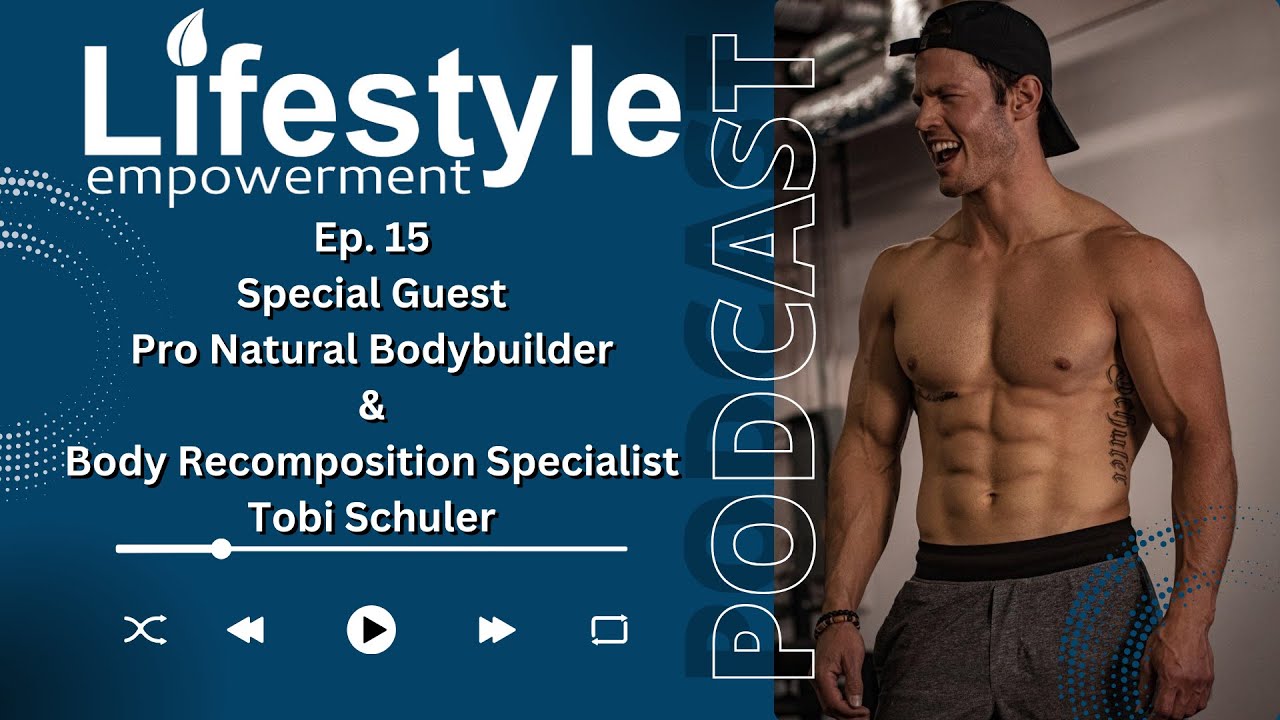This image appears to be a vertically-aligned rectangular advertisement for a podcast episode prominently featuring a muscular, shirtless bodybuilder named Toby Shuler. Toby, a pro natural bodybuilder and body recomposition specialist, is positioned on the right side of the image. He has a broad smile, a backward black baseball cap, visible tattoos along his chest and waist, a bracelet on his right arm, and is wearing gray sweatpants with a thick black waistband. On the left side, the background is dark blue, overlaid with a white block text reading "Lifestyle," with a leaf dotting the 'i.' Below that, "Empowerment" is written, followed by "Ep. 15," "Special Guest," and then Toby Shuler's professional titles. Additionally, there is a white line underneath his name, with a circular play button (a black triangle inside) and visible reverse and forward buttons, alluding to the interactive elements typical of a podcast player interface. The word "PODCAST" is also displayed vertically. The overall theme suggests an emphasis on fitness, motivating the audience towards weight training and body recomposition through the podcast.